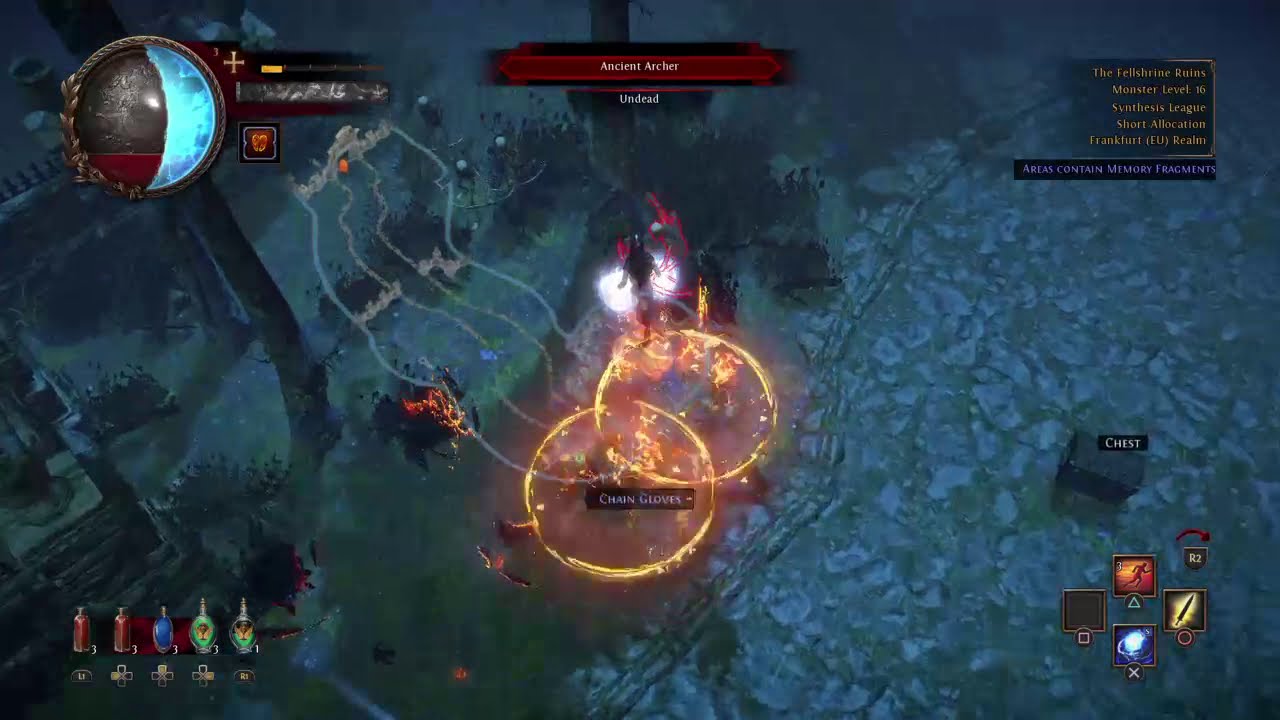This image is a detailed screenshot from the video game Path of Exile. The scene is viewed from a bird's-eye perspective and features a predominantly blue-gray, almost teal background. In the central portion of the image, a character is depicted levitating above two concentric, flaming rings, which emanate light and appear to include swirling streams of smoke. This central area is where the majority of the action happens, with the character and rings forming the focal point. 

At the top center, a red caption with white text reads "Ancient Archer" followed by "Undead," identifying the mob present in the scene. In the upper right corner, there is smaller, difficult-to-read text, referencing "areas contain memory fragments." The upper left corner displays a sphere or globe-like structure, featuring a crescent of blue on one side and darker shades on the other.

Moving to the lower regions of the image, the bottom left corner showcases various in-game elements like potions, bottles, and skills, while the bottom right corner includes an avatar and a chest, suggesting different in-game options or inventory items available to the player. The ground appears to be composed of stone, and the setting includes elements of an outdoor environment with visible trees and bushes.

Overall, this screenshot captures the adventurous and mystical ambiance of Path of Exile, emphasizing the central combat scene amidst an array of interactive gameplay elements scattered around the edges.